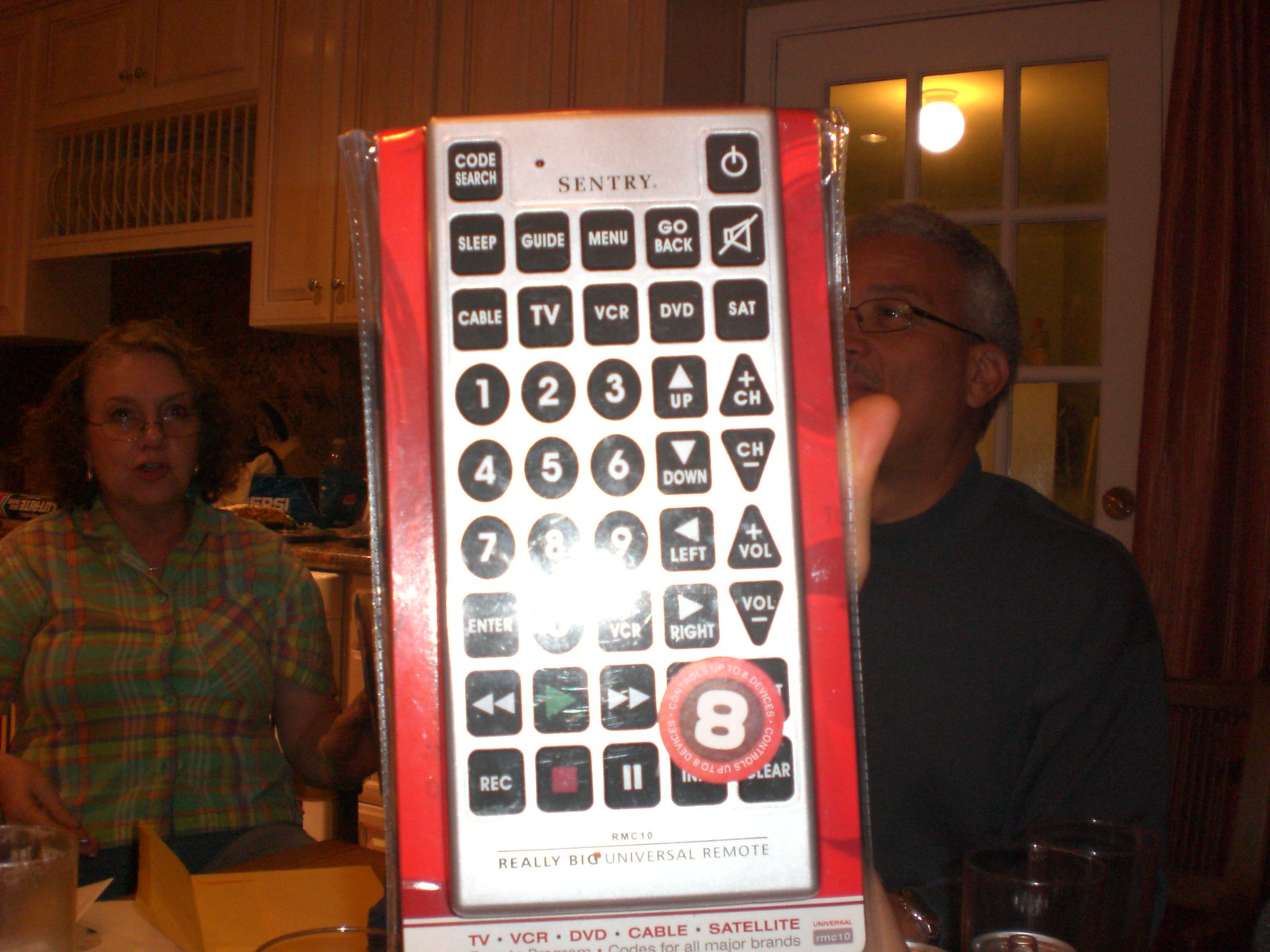The image features a man holding up a large, Sentry-brand universal remote control, wrapped in plastic that reflects the camera flash. The remote is silver with red sides and has a big number 8 sticker on it, suggesting multiple functionality modes. Bold letters at the bottom declare it as a "Universal Remote" suitable for TV, VCR, DVD, cable, and satellite for all major brands. In the background, the scene appears to be a home setting, possibly a kitchen, with cabinets, a door, and a light on, all bathed in a reddish glow. The man, who has salt and pepper hair and is wearing glasses and a black shirt, is holding the remote prominently in the center. To the left, a middle-aged woman with a multicolored plaid shirt featuring blue, yellow, and orange stripes appears to be speaking.